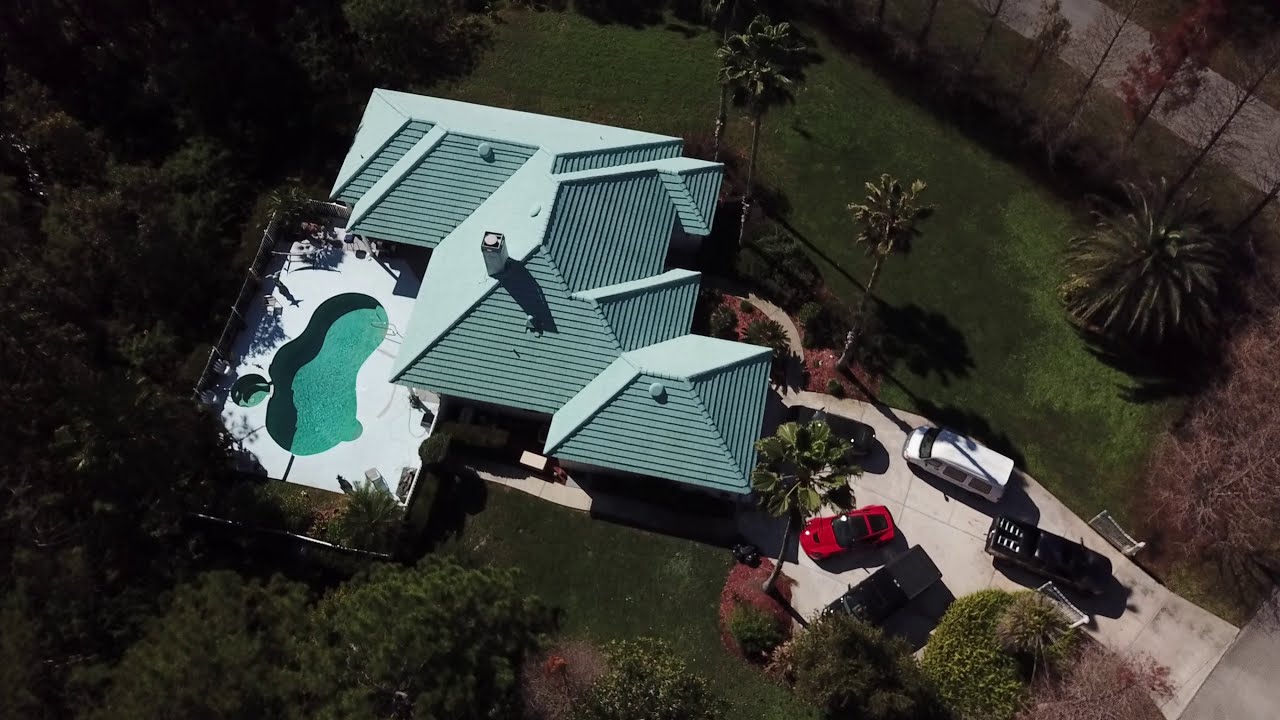This aerial view captures a large, upscale home situated slightly left of center in the image. The house features a pale blue, turquoise-like roof with multiple intersecting gables. To the left of the house, an irregularly shaped, kidney-like pool with teal-colored water is visible, accompanied by a circular hot tub to its left. Both the pool and hot tub are surrounded by a white, concrete patio. The right side of the image showcases a light-colored concrete driveway with four vehicles parked at various angles—two black cars, a red car, and a white van. The landscape is lush, with several palm trees prominently near the front of the house and a large green bush visible towards the top right. Dark green grass surrounds the property, enhancing the overall verdant atmosphere.